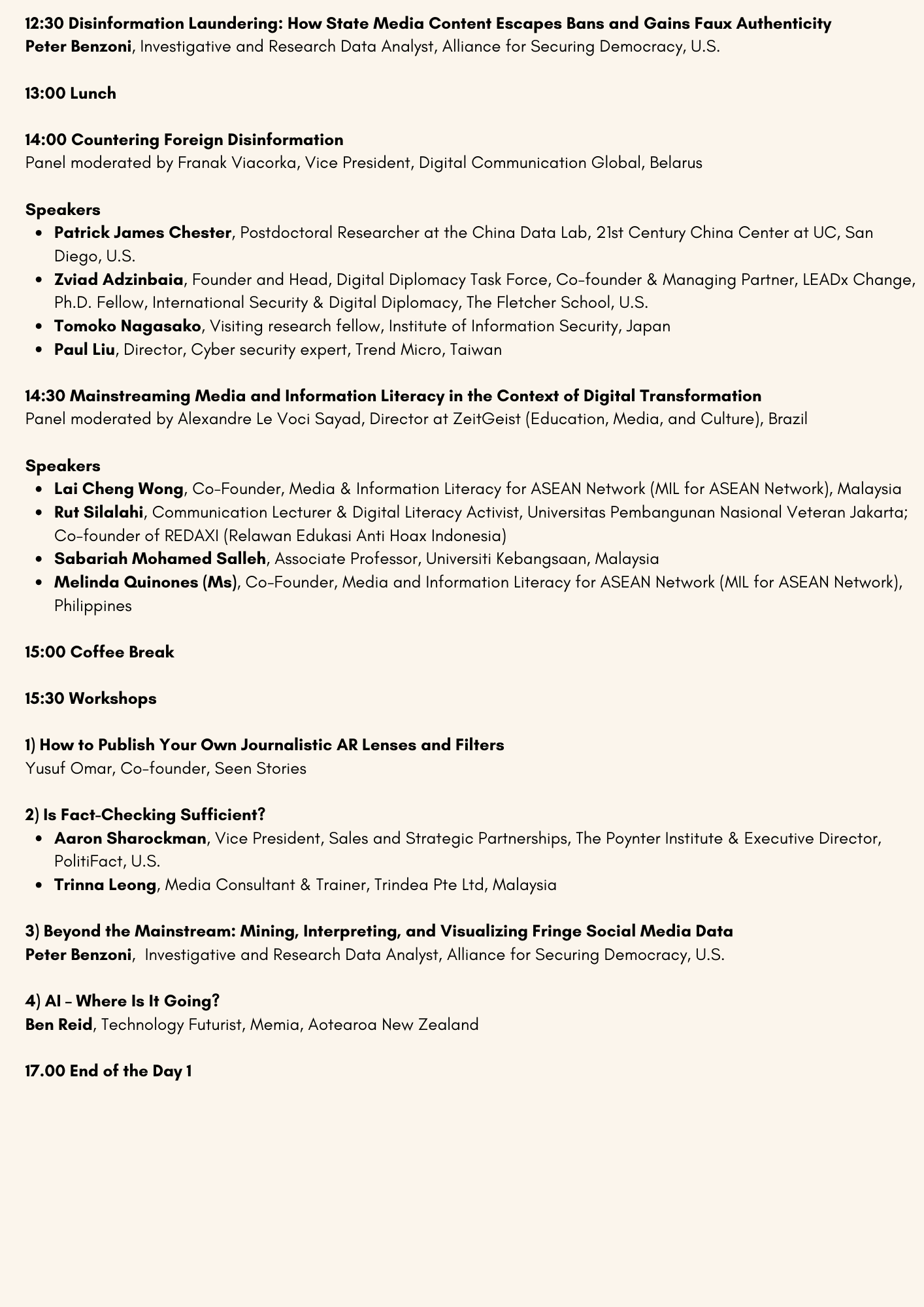### Event Schedule: Day One

**Time:** 12:30 PM - **Topic:** Disinformation Laundering  
**Description:** How state media content circumvents bans and gains faux authenticity.  
**Speaker:** Peter Benozzi, Investigative and Research Data Analyst, Alliance for Securing Democracy, U.S.

**Time:** 1:00 PM - **Lunch Break**

**Time:** 2:00 PM - **Panel:** Countering Foreign Disinformation  
**Moderator:** František Viačorka, Vice President Digital Communications, Global Belarus  
**Speakers:**
- Patrick James Chester, Postdoctoral Researcher at the China Data Lab, 21st Century China Center, UC San Diego, U.S.
- Zavod Od Zambia, Founder and Head of Digital Diplomacy Task Force, Co-founder and Managing Partner of Lead X Change, PhD Fellow in International Security and Digital Diplomacy, The Fletcher School
- Tomoko Nagasaka, Visiting Research Fellow, Institute of Information and Security, Japan
- Paul Lu, Director and Cybersecurity Expert, Trend Micro, Taiwan

**Time:** 2:30 PM - **Panel:** Mainstreaming Media and Information Literacy in the Context of Digital Transformation  
**Moderator:** Alexandre Livovichi Sayad, Director of Zeitgeist  
**Speakers:**
- Lei-Cheng Wong, Co-Founder, Media and Information Literacy of ACN Network
- Rout Silly, Communication Lecturer in Digital Literacy, Activist Universities Pembangonia Nasioni veteran Jakarta, Co-Founder at Redaxi
- Sabara Mohad Salih and Melinda Koneas, Co-founders, Media and Information Literacy at ACN Network

**Time:** 3:00 PM - **Coffee Break**

**Time:** 3:30 PM - **Workshops:**  
1. **How to Publish Your Own Journalistic AR Lenses and Filters**  
   **Facilitator:** Aaron Shaq Ruckman and Trina Leung  
2. **Is Fact-Checking Sufficient?**  
   **Facilitator:** Peter Penozzi, Investigative Research Data Analyst, Alliance for Securing Democracy  
3. **Beyond the Mainstream: Mining, Interpreting, and Visualizing Fringe Social Media Data**  
   **Facilitator:** Peter Penozzi, Investigative Research Data Analyst, Alliance for Securing Democracy  
4. **AI: Where’s It Going?**  
   **Facilitator:** Ben Reed, Technical Futurist, Memia, Atoria, New Zealand  

**Time:** 5:00 PM - **End of Day One**